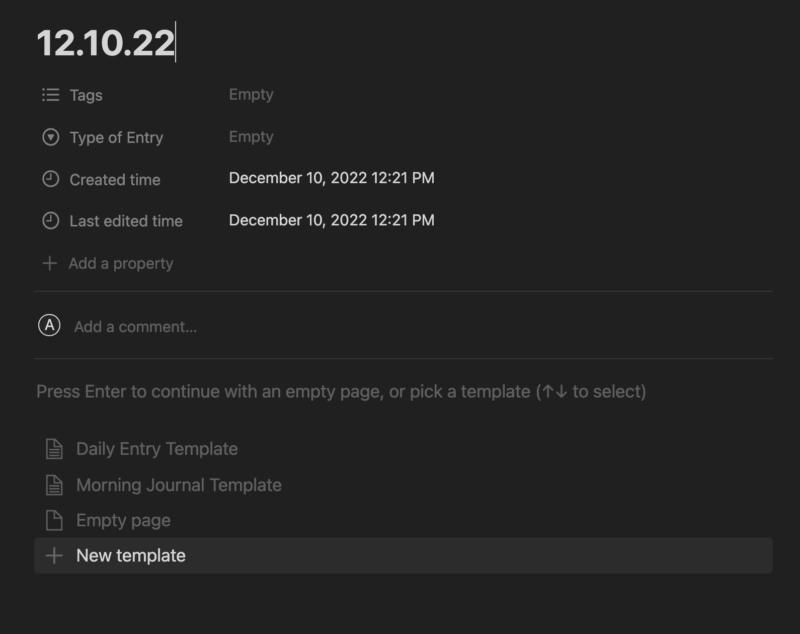**Screenshot of a Web Interface Capturing Tag and Template Entry**

The image displays a webpage with a tag and template entry section set against a minimalist black background. At the top of the interface, a date— "12 10 22"— is prominently displayed in white text. Below this, three horizontal lines adjacent to the word "Tags" are shown; a few tabs over, the field is marked as "empty," adorned with a down-arrow icon inside a circle labeled "Type of Entry," which is also empty.

Directly beneath, a clock icon appears next to the label "Created Time," indicating the timestamp as December 10th, 2022 at 12:21 PM. Another clock icon below it denotes "Last Edited Time," reflecting the same timestamp. Following this, a plus sign is present alongside the instruction "Add a Property," with a note that no properties have been added yet.

Centrally located on the page is a subsection indicated by a circular "A" icon paired with the text "Add a Comment," currently blank. An instruction reads, "Press Enter to continue with an empty page or pick a template," with a hint in parentheses mentioning to use up and down keys to select.

Lower down, several paper icons represent different template options. The first icon is labeled "Daily Entry Template," followed by another labeled "Morning Journal Template." The subsequent icon signifies an "Empty Page." The final element is a highlit plus sign contained within a grayer box and white font, labeled "New Template."